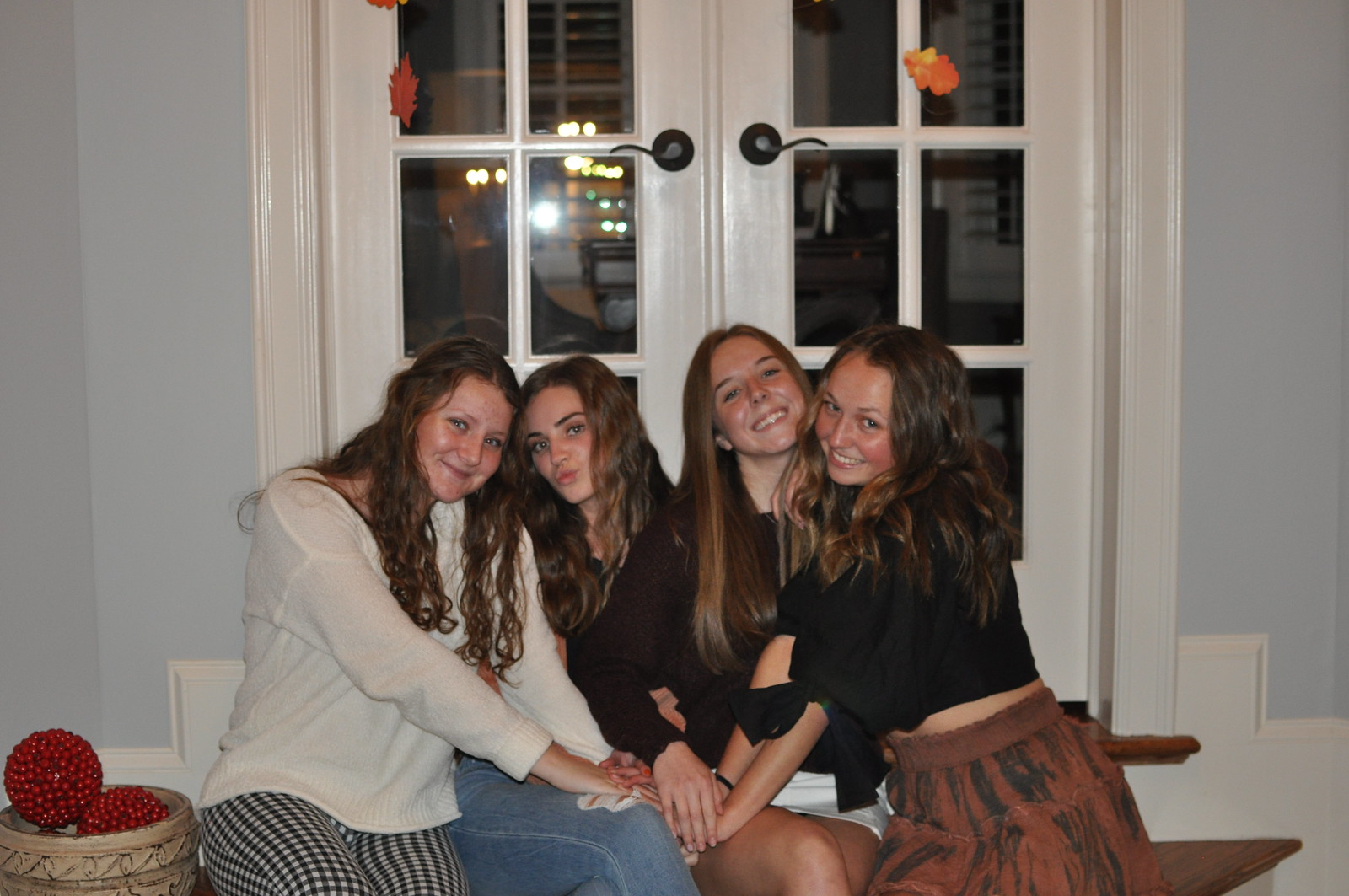The image captures four pre-teen to teenage girls, all seated closely together on a step in front of glossy white French double doors with black handles and decorated with fall-themed orange leaves. The backdrop features light blue or possibly gray walls. The girls are embracing each other warmly, either smiling or making playful faces. 

From left to right, the first girl, with wavy brown hair and a white sweatshirt, sports black and white patterned pants. The second girl, also with wavy brown hair, wears navy blue jeans and a black shirt, her lips pursed in a playful kiss. The third girl, with straight brown hair, dons a short white skirt and a black shirt. The fourth girl has wavy brown hair, a black shirt, and a burnt orange patterned skirt. Beside them, on the left, is a beige ceramic urn containing decorative red balls made from small beads. The ambiance suggests an autumn setting, echoed by the leaf decorations and the warm, cozy clothing.